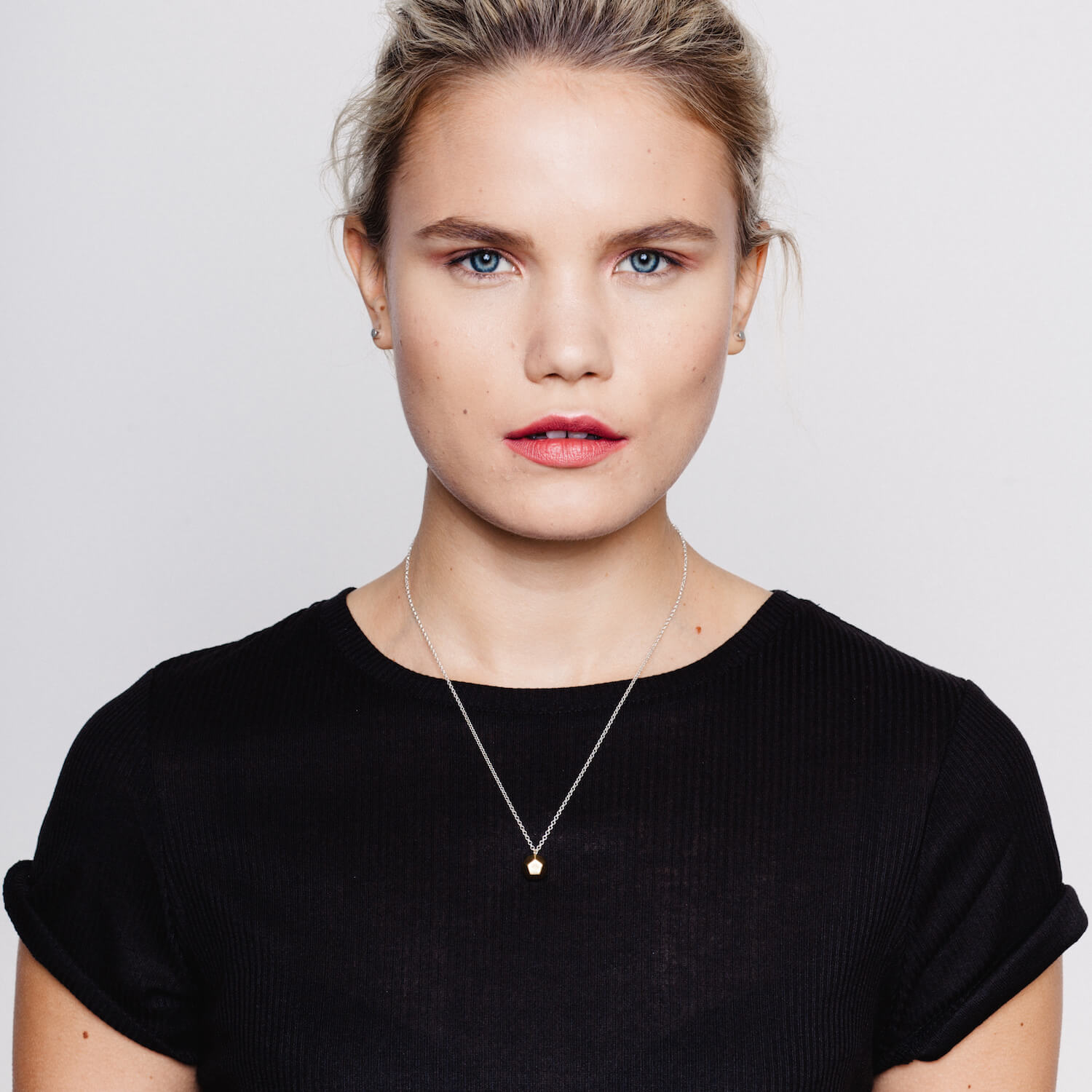The image features a young woman, posed and staring directly at the camera against a white background. Her blonde hair, accented with brown highlights, is pulled back, showcasing a few baby hairs along the sides of her face. She has pronounced, bushy eyebrows of a dirty blonde or light brown hue, framing her deep blue, hooded eyes. Her cheeks are contoured, providing a slight shadow. She wears lipstick in a light reddish-pink shade, with her two front teeth peeking through partly open lips. Her outfit consists of a plain black short-sleeved T-shirt with rolled-up sleeves that expose her arms, and the shirt appears slightly gauzy, revealing a black bra underneath. Adorning her neck is a thin silver necklace with a small circular pendant, likely featuring a diamond. Completing her look are small diamond stud earrings in each ear. Her skin is fair, and her plain, posed demeanor suggests this could be an advertisement for either the clothing or the jewelry she wears.